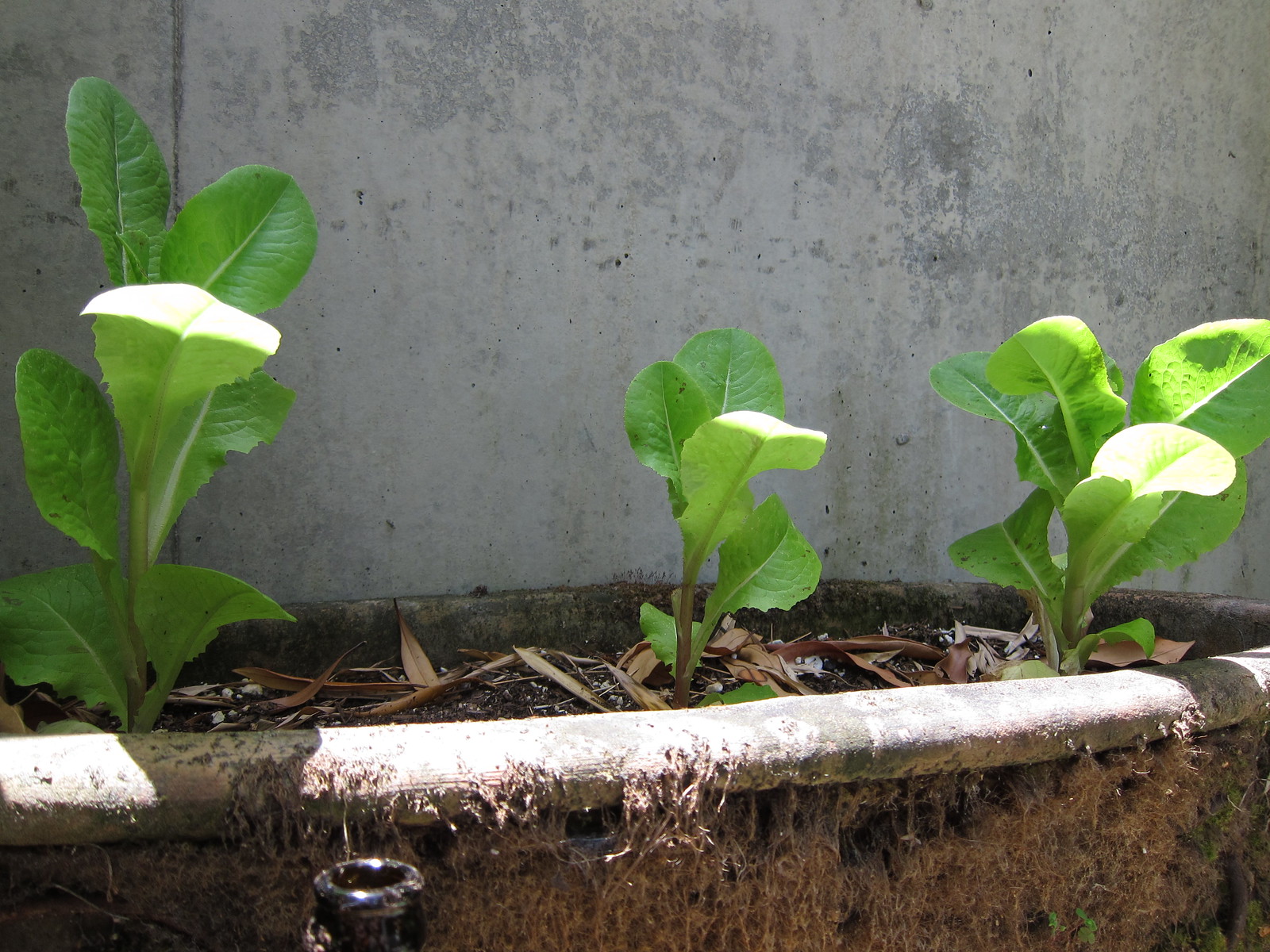The image showcases an outdoor scene featuring a weathered concrete wall with varying shades of gray, including darker splotches. In the center foreground, there's a large, visibly dirty flower pot with a gray rim and a brownish body. Near the bottom of the pot, a black object with a noticeable opening can be seen, possibly an old beer bottle. The pot is filled with dirt and sprouting plants. There are three distinct plants: one on the far left with green leaves that clearly display their veins and a bent white-tipped leaf, another positioned slightly right of center, smaller but also with a white-tipped bent leaf, and a fuller plant on the far right showing lighter green spots. The scene is brightly lit by the sun, casting shadows on the concrete ridge and adding depth to the image.